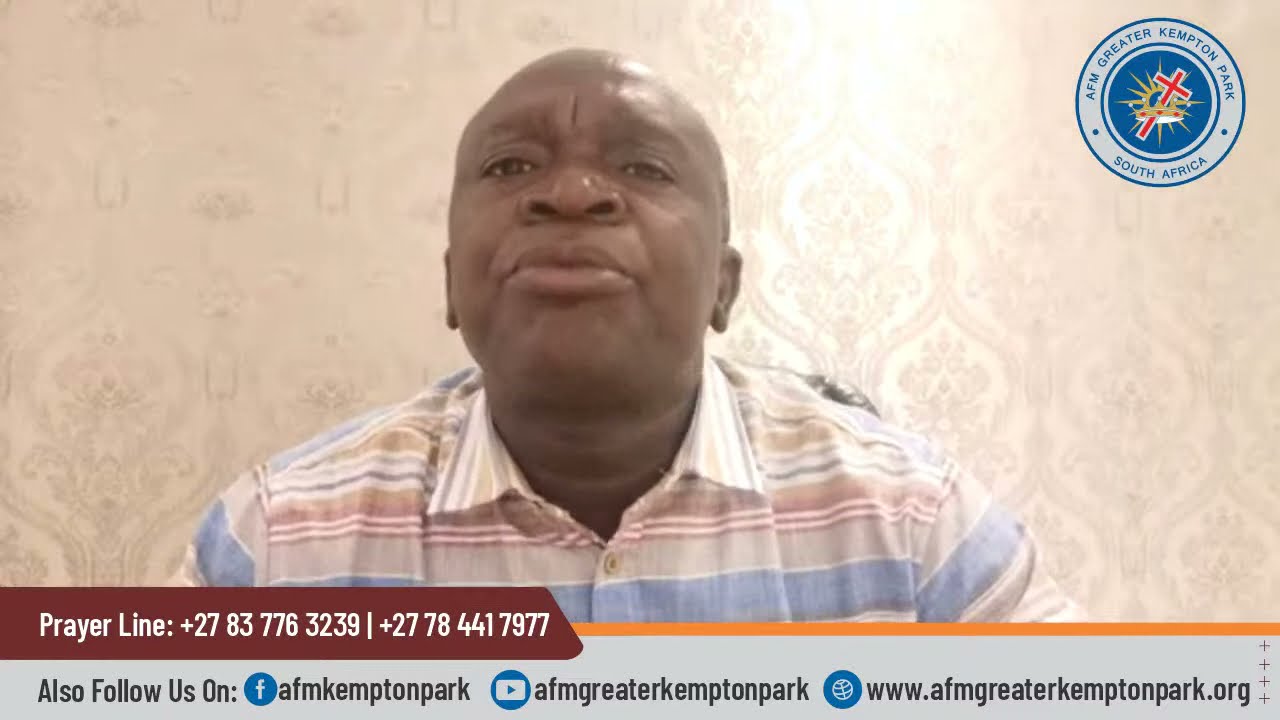The image is a screen capture likely from a television broadcast of a church service or advertisement for the AFM Greater Kempton Park in South Africa. It features a central figure—a bald African-American man with a serious expression, gazing slightly upward with pursed lips, possibly in mid-speech. He is wearing a vividly striped, collared shirt with colors including orange, gray, red, yellow, white, and blue. The backdrop is a decorative, light-colored wallpaper with a mandala pattern. In the top right corner, there's a logo depicting a cross with a crown and rays of sunlight, labeled "AFM Greater Kempton Park, South Africa." The bottom portion of the screen displays a red banner labeled "prayer line" along with contact numbers: +27 83 776 3239 and +27 78 441 7977. Furthermore, it prompts viewers to follow them on Facebook at "AFM Kempton Park," includes a YouTube icon, and provides a web address: "www.afmgreaterkemptonpark.org."